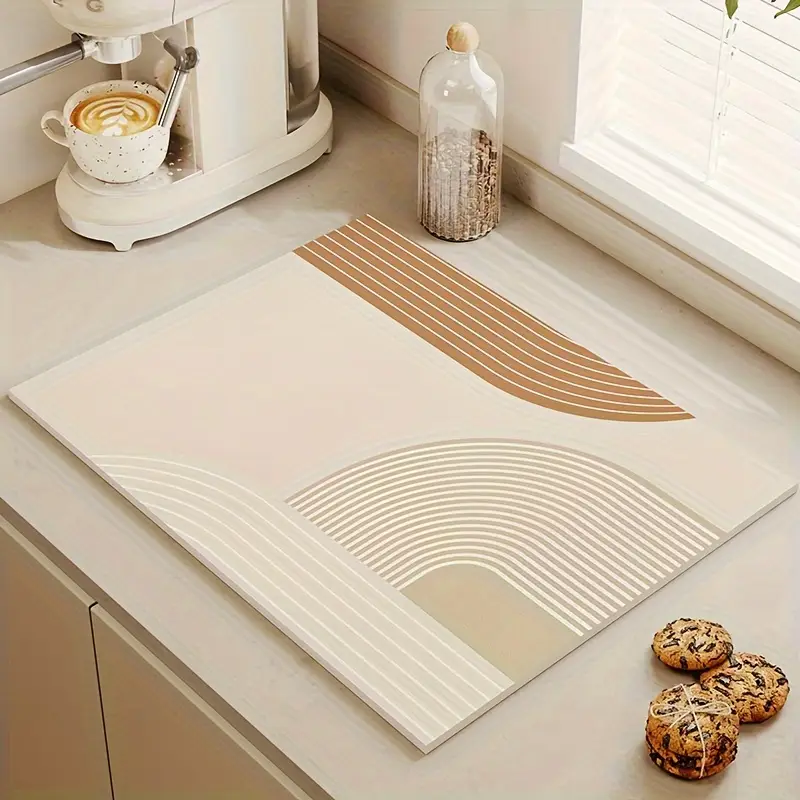In this image, we are looking at a tidy kitchen countertop positioned in front of a window with white mini blinds partially open, allowing sunlight to filter through. The countertop is pristine white and features a pad or mat with a rectangular design on it, possibly indicating an inductive stovetop cover. To the right of this mat, there are three chocolate chip cookies, one of which is stacked with a piece of string tying three cookies together, while two more rest just above the stack.

On the left side of the image, an espresso maker sits at the end of the counter. The machine is equipped with a foamer, and there's a cappuccino cup positioned underneath. The cup is white and adorned with speckles, holding a cappuccino that features an artistic leaf design in the foam.

Adjacent to the coffee machine and closer to the padded mat, a glass bottle with a cork top is visible. The bottle contains small pebbles or possibly walnuts, adding a rustic touch to the scene. This kitchen setup, while minimal, exudes a warm and inviting atmosphere, perfect for a relaxing coffee break.